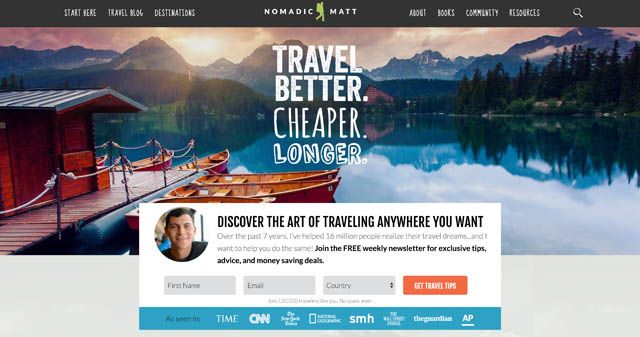The image showcases a scenic website with a layout that is approximately one and a half to twice as wide as it is tall. At the top, there is a black background spanning about five to ten percent of the image’s height, adorned with white text overlays presenting the site’s navigation menu. On the left, the menu options include "Start Here," "Travel Blog," and "Destinations."

Centrally positioned, the website’s logo features "Nomadic Matt" in bold, white capital letters. Nestled between these words is a lime green silhouette of a backpacker facing right. Moving to the right side of the menu, you find additional options: "About," "Books," "Community," "Resources," and a magnifying glass icon for search functionality.

Directly below the navigation bar lies a visually captivating banner. The banner shows a serene lakeside scene with idyllic features. On the left, there’s a quaint hut and dock, surrounded by several wooden rowboats. The calm lake perfectly reflects the picturesque surroundings, doubling the beauty of the landscape which appears to be set against a backdrop of mountains either at sunrise or sunset.

At the bottom of this banner, there is an overlay featuring a profile picture accompanied by a compelling call to action, “Discover the art of traveling anywhere you want.” Below this text, the site prompts users to enter their first name, email, and country, followed by a button inviting them to get travel tips.